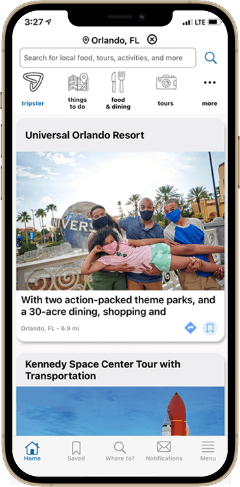This image showcases an iPhone, identifiable by its signature design and hardware features. On the top left side of the device, there is a switch to silence the ringer. Below this switch are the volume up and down buttons. On the right side of the phone, the power button is visible. The screen of the iPhone displays a resort booking app with a search bar at the top, where "Orlando, Florida" is typed. Immediately beneath the search bar are several navigation tabs labeled "Tripster," "Things to Do," "Food and Dining," "Tours," and "More." 

The main part of the screen features detailed listings. The first listing displays "Universal Orlando Resort" with an image of people celebrating and posing for pictures. Accompanying this image is text that begins with "With two action-packed theme parks and 30 acre" but is truncated. The second listing is titled "Kennedy Space Center Tour with Transportation," featuring a picture of a rocket. The clean and organized interface of the app aims to offer a user-friendly experience for booking and exploring various travel options in Orlando, Florida.